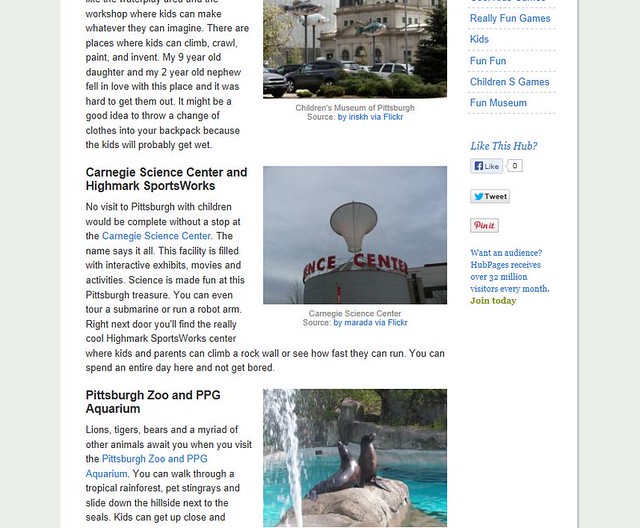**Captivating Spots for Families in Pittsburgh: A Visual and Informative Guide**

This engaging image-based guide offers an immersive overview of various family-friendly attractions in Pittsburgh. The upper portion of the image features vibrant text that introduces a workshop at the Children's Museum of Pittsburgh, emphasizing its creative and interactive environment. The narrative highlights areas where kids can climb, crawl, paint, and invent, making it a haven for exploration and imagination. A personal touch is added with a mention of the creator's nine-year-old daughter and two-year-old nephew, who both adored the place so much that leaving was a challenge. A practical tip is offered to parents, advising them to pack a change of clothes due to the likelihood of kids getting wet.

Prominently displayed is a photo of the museum, captioned with the establishment's name, sourced by Irish via Flickr.

Adjacent to this, there's information on the Carnegie Science Center and Highmark Sports Works. The text suggests that a visit to Pittsburgh with children isn't complete without stopping here, noting the facility's wealth of interactive exhibits, movies, and activities that make science entertaining. Highlights include the opportunity to tour a submarine and operate a robot arm. Additionally, the nearby Highmark Sports Works Center provides exciting physical activities like rock climbing and sprint challenges, ensuring a day's worth of fun for both kids and parents. Accompanying this section is an image of the Science Center, easily recognizable with its bold red lettering and a distinctive large white circular structure atop the roof.

Further down, the page delves into the wonders of the Pittsburgh Zoo & PPG Aquarium. This section describes an array of animals, including lions, tigers, and bears, alongside the interactive experiences the zoo offers, such as walking through a tropical rainforest, petting stingrays, and sliding down a hillside next to the seals. The visual aid here depicts animals perched on rocks within a watery habitat.

The overall layout of the image features a clean design, with a white background, black text, and subtle gray borders, ensuring that the content remains clear and visually appealing.